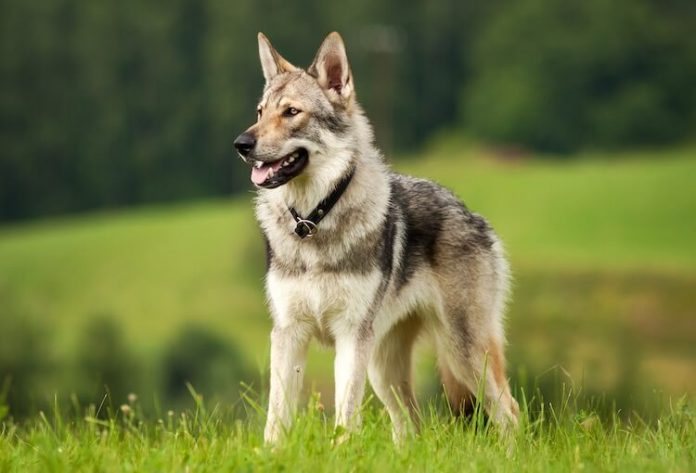This image features a dog with a strikingly lupine, or wolf-like, appearance, captured in a three-quarter view. The dog is gazing to the left with ears pointed straight up, exuding an alert and interested demeanor. Its mouth is slightly open, revealing a glimpse of its teeth and tongue. The coloration of the dog is a mix of beige, tan, brown, black, white, and gray, giving it a rich, variegated coat. Around its neck, it wears a black collar that fits loosely. The backdrop consists of a bright green grassy area, with dark, blurry trees or bushes visible far in the distance. The dog's stance appears natural and relaxed, as it stands amid the serene outdoor setting.